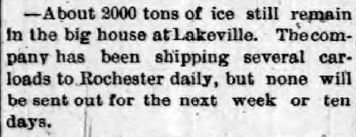The image features a small, rectangular newspaper clipping, seemingly a digital scan that shows signs of age and digital artifacting, such as light gray tones and scratch marks. The clipping has a slightly dingy white background with black text in old typewriter font, indicating it was likely scanned from an old newspaper. The text itself starts with a hyphen and reads: "About 2,000 tons of ice still remain in the big house at Lakeville. The company has been shipping several carloads to Rochester daily, but none will be sent out for the next week or 10 days." There are no other writing or identifiable markers, such as a date, on the clipping.